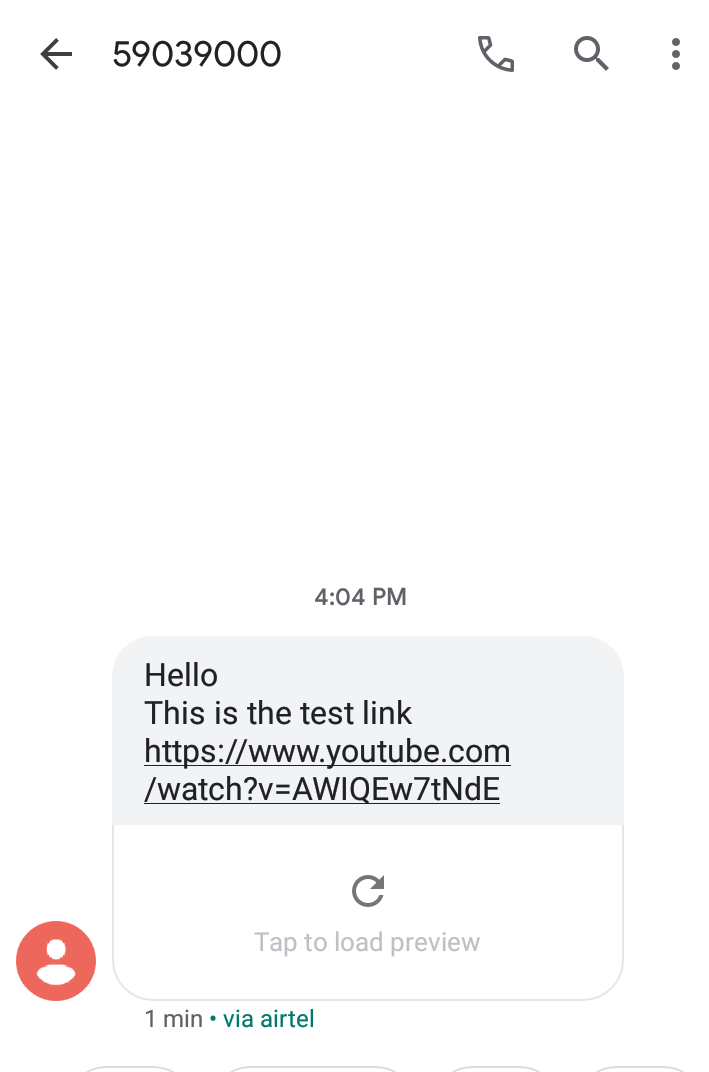Screenshot of a test link for my cell phone. The background is primarily white, with the top left corner featuring a black directional arrow pointing to the left. Following the arrow is a string of black text displaying "59039000." To the right, there is a handset phone icon, a black magnifying glass icon, and three vertical dots in succession. Below this section is a large empty white space.

Centered beneath the white space, in a lighter black or charcoal black text, is the time "4:04 p.m." Further down, there is a rectangular box with rounded corners. The top half of this box is light gray, containing black text that reads: "Hello, this is the test link: https://www.youtube.com/watch?v=awiQew7tnde." The URL is underlined for emphasis.

Beneath the light gray section is the bottom half of the box, which is white. Inside the white section, there is a circular directional arrow. Below this arrow, it reads: "Tap to load preview."